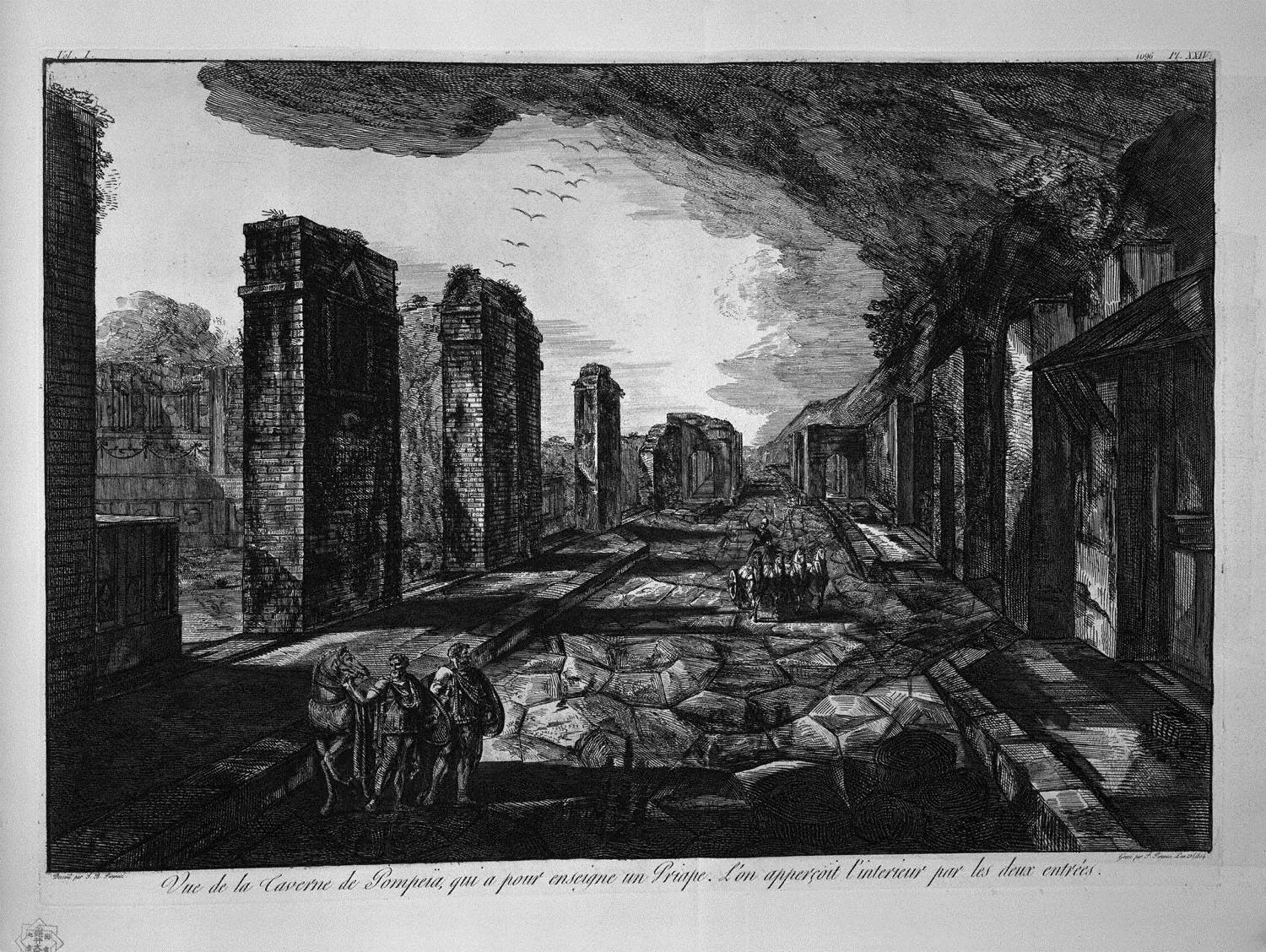The artwork is a highly detailed, black-and-white sketch or possibly a charcoal or woodblock print depicting a dramatic, ancient scene. The image showcases a fractured stone roadway that appears to traverse a broken-up bridge or a dilapidated old-world street, lined with imposing columns and brick walls that suggest the remnants of ruins. Adding to the historical atmosphere, plants are seen growing amidst the destruction. The sky above is dominated by dark, ominous clouds, contrasting sharply with birds flying through the brighter sections of the sky.

On the left side of the scene, two tall men, likely warriors, stand beside a horse, one of them equipped with what looks like a large shield. Their presence hints at the possibility of concealed weapons. Further down the road, a chariot drawn by four horses is visible, suggesting a Roman era as confirmed by figures dressed in robes. Shadows and an overall somber tone pervade the illustration, with the exception of the relatively bright sky. Text inscribed at the bottom, partially readable, includes the word "Pompeii," hinting at the historical and geographical context of the scene.